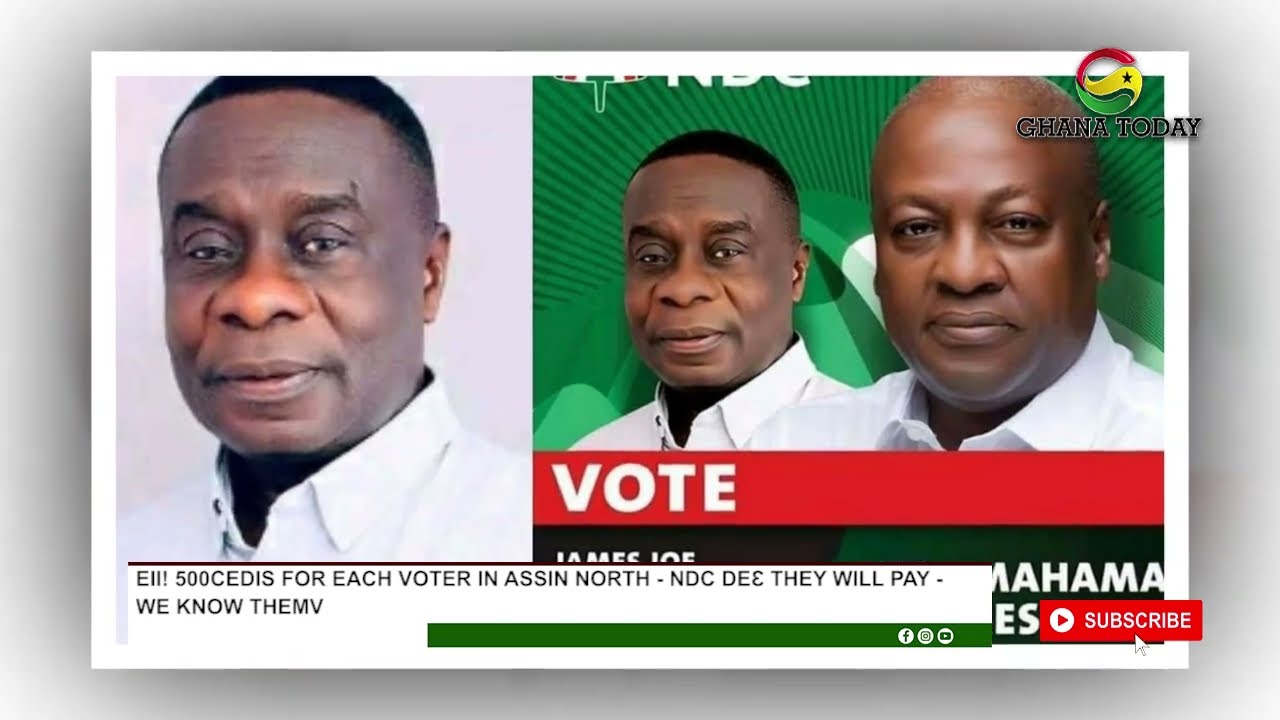The image is a detailed poster featuring a call to vote, with a composition divided into two main sections. On the left side, there is a close-up of a black man with short black hair, wearing a white collared shirt over a darker shirt, set against a tan background. On the right side, the same man appears again, standing next to another black man who is similarly dressed in a white collared shirt, both set against a green background. Above everything on the top right, the words "Ghana Today" are prominently displayed, suggesting a network or website affiliation. Beneath the men on the right side, text in white letters on a red banner urges, "Vote James Joe." At the bottom of the image, additional text reads, "500 CEDIS for each voter in Assin North - NDC - DE." Further, it states, "They will pay. We know them." A green bar runs across to the right, accompanied by a red subscribe button, adding a digital or broadcast element to the poster. The color palette includes tan, green, white, black, red, and yellow, enhancing the visual contrast and emphasis on the electoral message.